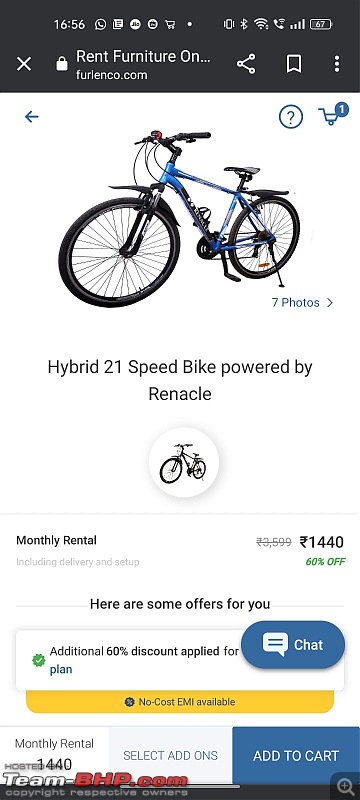This image is a mobile device screenshot showcasing a webpage from furthenco.com, a bike and furniture rental service. The device's status bar displays standard icons, including the current time, WhatsApp notifications, Bluetooth and Wi-Fi connectivity, and battery status. The webpage prominently features a single product: a blue Hybrid 21-speed bike powered by Renault Core. Detailed information about the bike's monthly rental cost is provided, listed at 1,440 in the local currency. Additionally, the page highlights a special offer, showing that the current rental plan enjoys a 60% discount. Options for selecting various add-ons and offers are also visible at the bottom of the screen.